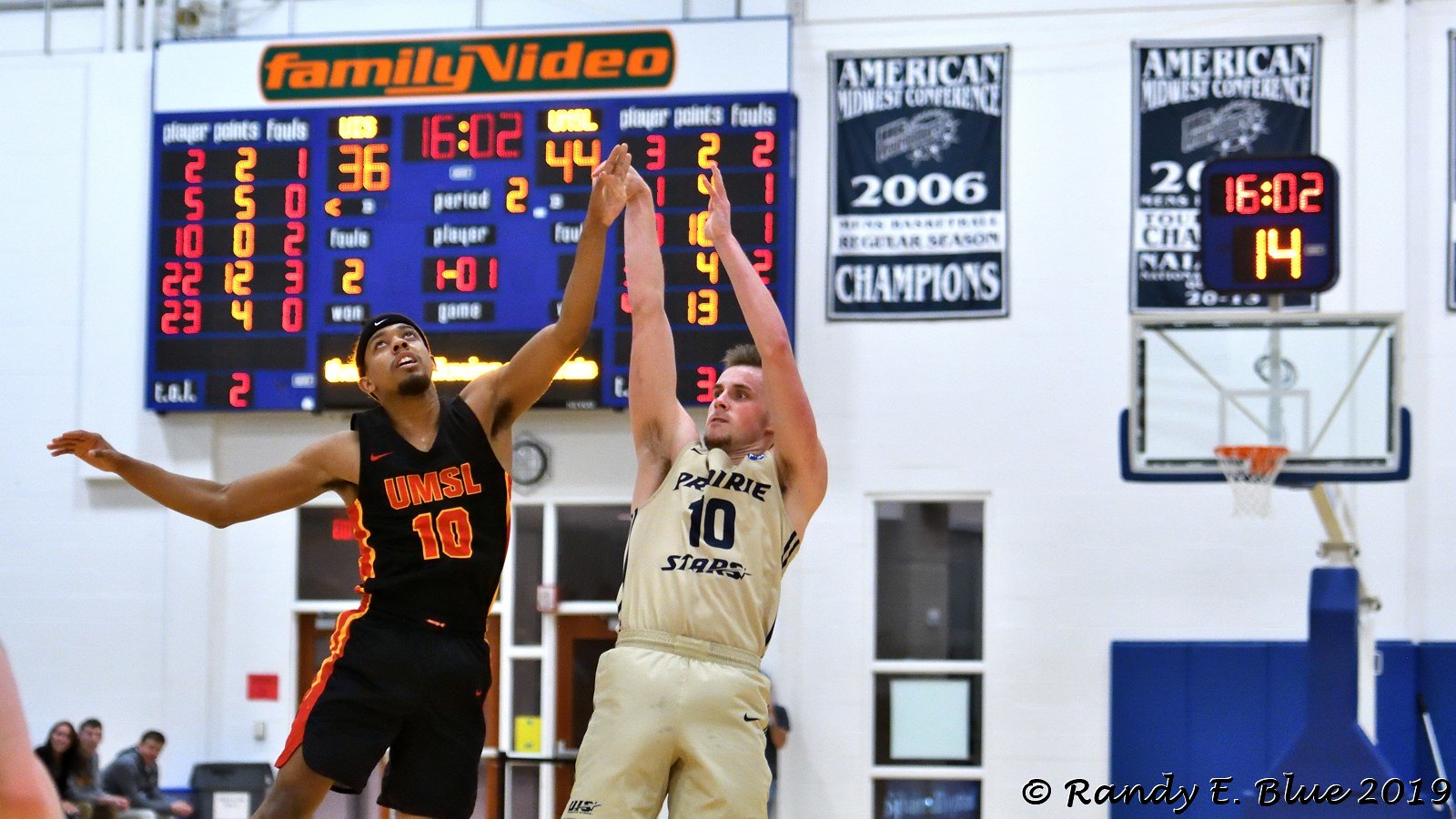The image features two basketball players, a black man on the left and a white man on the right, both airborne with arms raised, seemingly reaching for an unseen ball. The black player, wearing black shorts and a black jersey with "UMSL" and number 10, contends with the white player, who is clad in a white uniform with "Prairie Stars" and also sporting the number 10. In the background, a scoreboard prominently displays "Family Video" in orange letters on a green banner, detailing various scores in red and orange. Above the scoreboard, championship pennants are visible, indicating titles from the American Midwest Conference Champions in 2006 and another partially obscured year. The game, as captured by Randy E. Blue in 2019, shows spectators on the lower left, while the general background is mostly white walls accented by the scoreboard and banners.